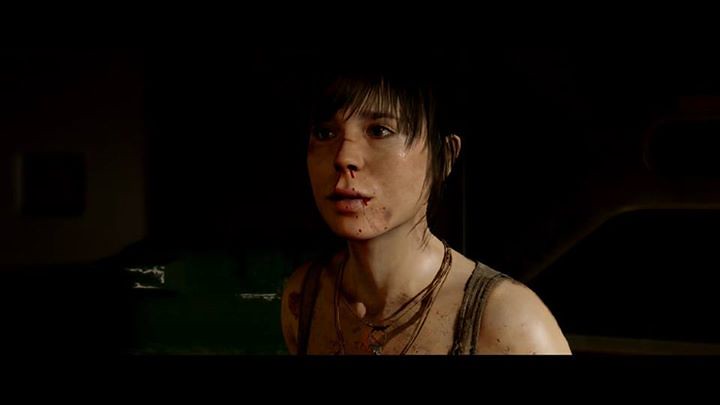The image, likely from a horror-themed video game, depicts a Eurasian woman at the center, emitting an unsettling aura. She showcases a distressed appearance, marked by a nosebleed and a bloodied lip. Her attire includes a tribal necklace resting prominently against her chest, and a tank top that reveals a significant amount of skin. Her black hair is styled with some bangs cascading over her forehead, lightly exposing her left ear. The character stands against a backdrop of nearly complete darkness, intensifying the eerie and grim ambiance of the scene.